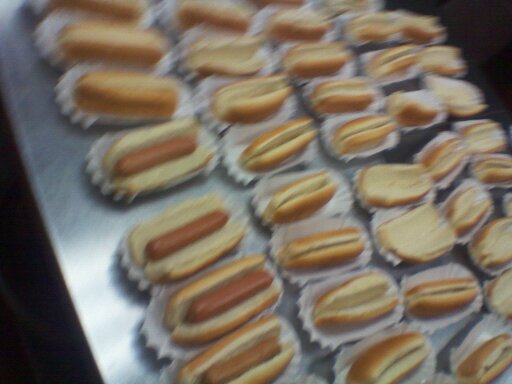This slightly blurry photograph captures a collection of hot dogs and buns arranged on a slick stainless steel table. In the foreground, a row of hot dogs in buns is neatly lined up, each nestled in frilly paper holders typically used at sporting events like baseball games. Behind this row, there are four more rows consisting solely of empty, open buns. The arrangement appears somewhat uneven, with the buns in various states of openness. The background features a black spot in both the upper right and lower left corners. In total, there are around 30 buns, though precise counting is hindered by the blurry nature of the image.